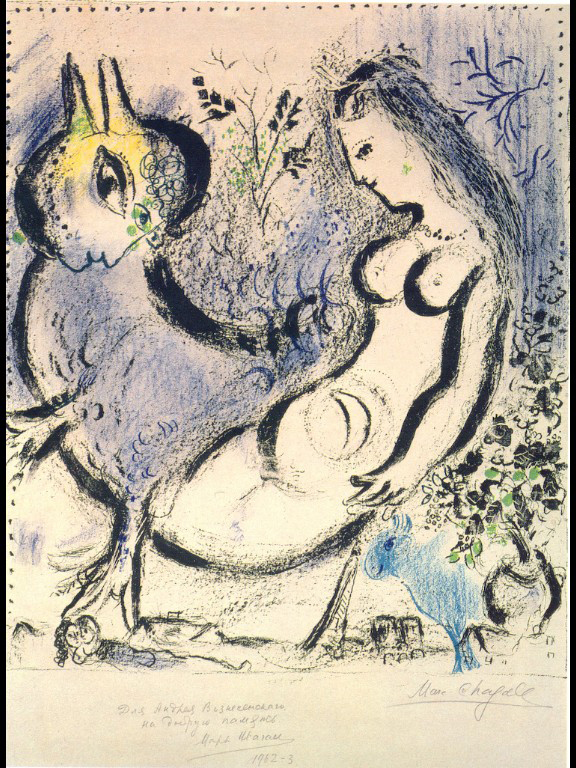This image is a highly detailed artwork on a white sketch pad, depicting an abstract and surreal fusion of a partially nude woman and a bird. The woman, with long black hair, is facing left with her head tilted downward, her left arm resting at her side while her right arm is not visible. Her bare chest is prominently displayed, and the lower portion of her body seamlessly transitions into a large, mythical bird. The bird is blue with a yellow beak, a big blue eye, and claws. The artistry is further complemented with green leaves scattered around, giving a lively touch to the surrounds.

Additionally, intricate elements such as flowers, a vase with a plant on the far right, and multiple floating leaves add depth to the scene. Near the bottom of the artwork, there's a small sketch of two figures connected to each other, one of which resembles a Howdy Doody-like character, smirking while lying down. A moon is drawn on the woman's stomach, enhancing the whimsical feel of the piece. The artwork is bordered by a thick black line and marked with the date "1982-3" at the bottom. There is also some indistinct writing next to the date, and visible pencil markings, suggesting it was made with markers, crayons, and colored pencils.